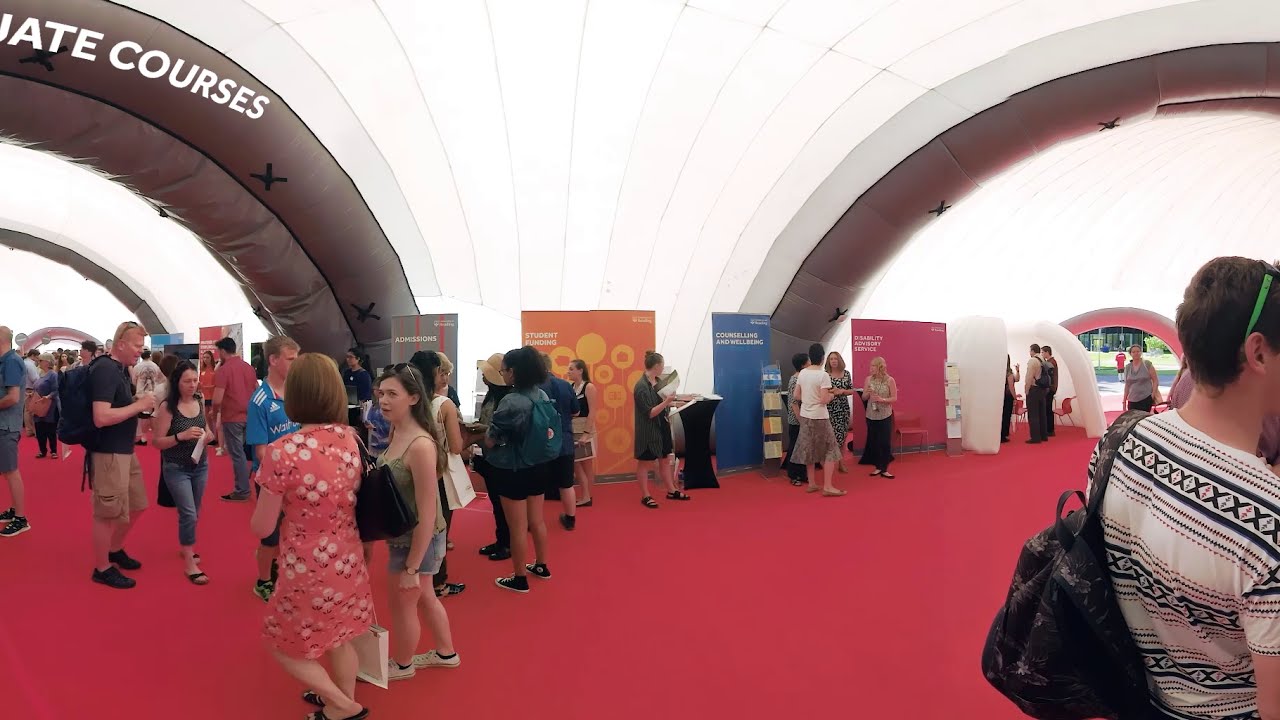The image captures a vibrant and bustling interior of a large, air-inflated tent resembling a convention hall. The tent's structure is strikingly curvaceous, with white fabric accented by brown trimmings that create a column-like effect on the roof, giving it a distinct "bubbly" appearance. The floor is entirely covered with a bold red carpet. Throughout the space, numerous people, dressed casually and carrying bags or backpacks, are seen milling about. 

Bright daylight filters through, illuminating the scene with a natural brightness. Positioned against the rear and edges of the tent are multiple colorful signages in hues of orange, blue, red, and gray, displaying phrases such as "student funding," "counseling," "well-being," and partly visible "ATE Courses," suggesting an educational or college recruitment context. A noticeable archway on the right side serves as an entrance and exit, with a constant flow of attendees moving through it. The overall image is crisp and clear, with a wide spectrum of colors like green, yellow, and black, adding to the engaging and dynamic atmosphere of the event.